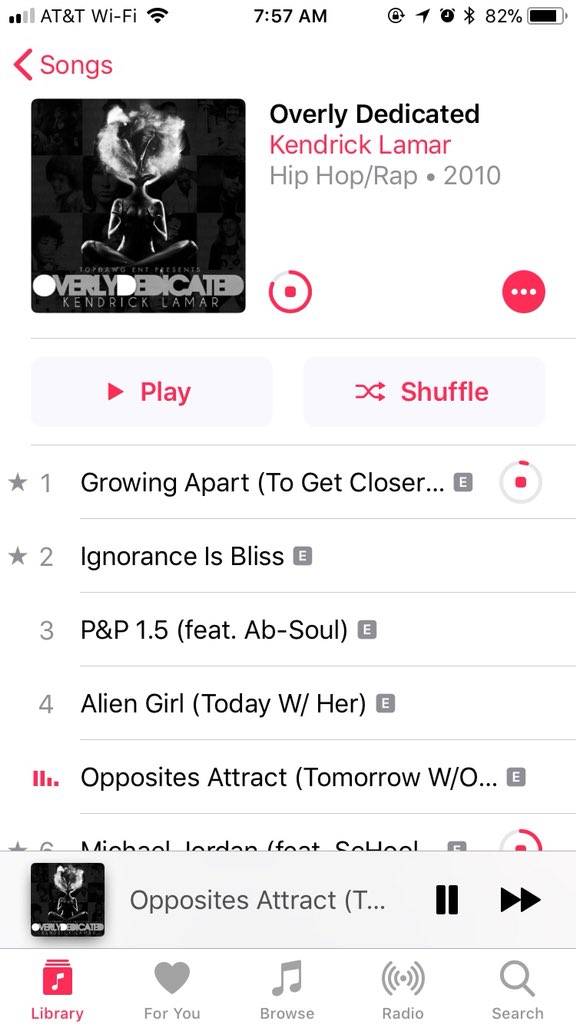This screenshot displays a mobile device screen at 7:57 AM, connected to AT&T Wi-Fi with the battery level at 82%. The focal point of the image is the album cover for Kendrick Lamar's "Overly Dedicated," released in 2010, categorized under Hip Hop and Rap. The album cover features an image of a female sitting with her legs crossed. Music playback controls are visible, including a play button and a shuffle button. The tracklist is partially visible, highlighting:

1. "Growing Apart (To Get Closer)" — marked with a star.
2. "Ignorance Is Bliss" — marked with a star.
3. "P&P 1.5" featuring Ab-Soul.
4. "Alien Girl (Today With Her)."
5. "Opposites Attract (Tomorrow)."
6. "Michael Jordan" — marked with a star.